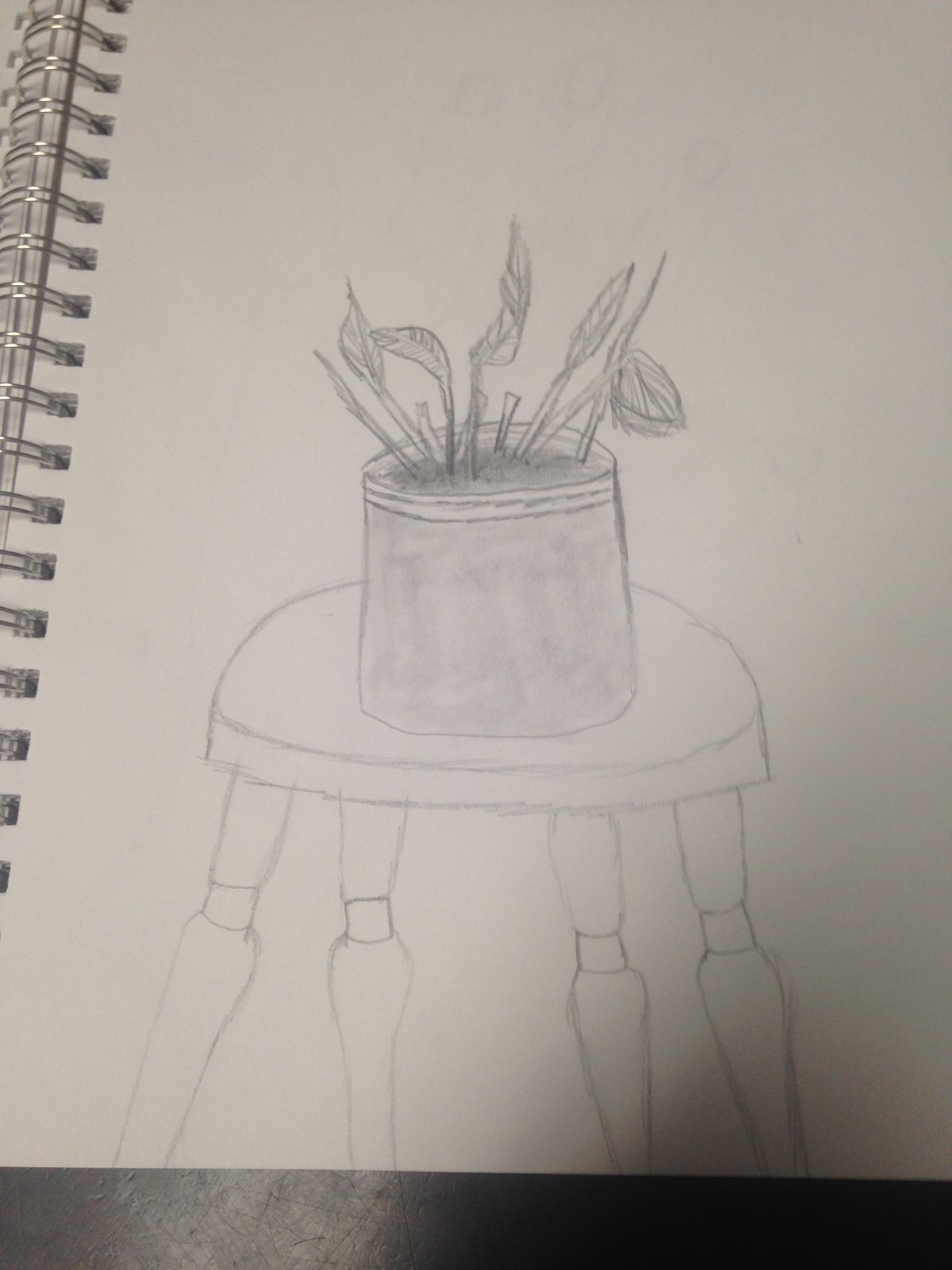The image showcases a detailed pencil sketch on spiral-bound notebook paper or a sketch pad. The drawing features a round table with four legs, depicted without any color. Atop the table rests a medium-sized planter containing sprouts with small leaves, approximately seven in total. The leaves and soil within the planter are subtly shaded in black. The composition suggests an amateur style, yet it captures the essential details well. The sketch is set against a backdrop that includes part of the metal or dark-colored table where the notebook is laid open. The silver spirals of the sketchbook are visible on the left side, reflecting light. Additionally, the viewer's shadow is faintly discernible in the bottom right corner of the photograph.